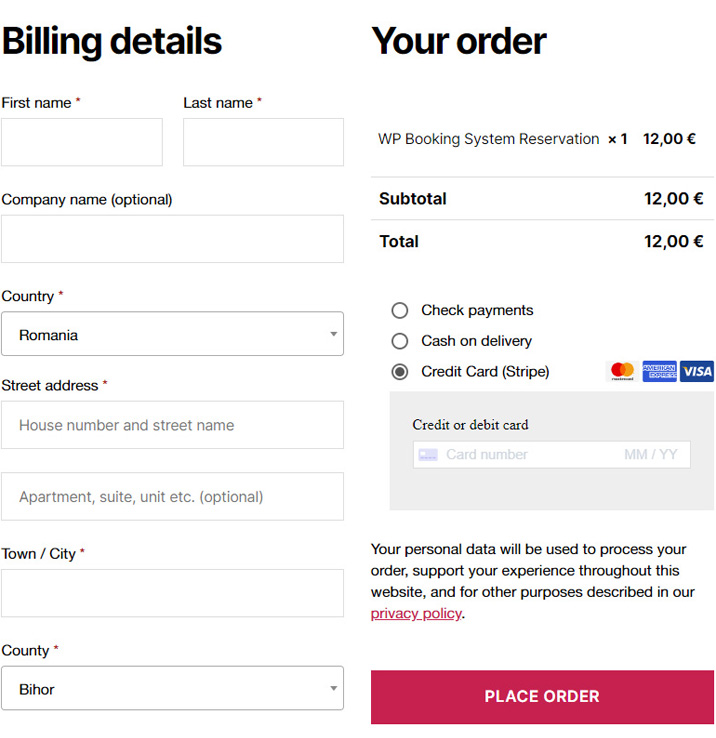The image depicts a section of an online checkout screen, where a user is in the process of completing an order. On the left side of the screen, under the header "Billing Details," various fields are displayed for the user to fill in, including First Name, Last Name, Company Name, Country, Street Address, Town/City, and County. All fields are currently empty, except for the "Country" field, which is populated with "Romania." The "Street Address" field is divided into two smaller fields: the first for the house number and street name, and the second for additional details such as apartment, suite, or unit number.

To the right of the "Billing Details" section, there is a summary labeled "Your Order." It lists the item as "WP Booking System Reservation" at a cost of 12 euros, which is also the subtotal. Below this summary, the user must select a payment method. In this instance, the payment method chosen is "Credit Card (Stripe)." 

Beneath the payment selection, there is a field for entering credit card information, including the card number and expiration date (month and year). Further down, a privacy statement informs the user that their personal data will be used to process their order, support their experience on the website, and for other purposes as outlined in the privacy policy. At the very bottom of the screen is a button labeled "Place Order," which finalizes the transaction.